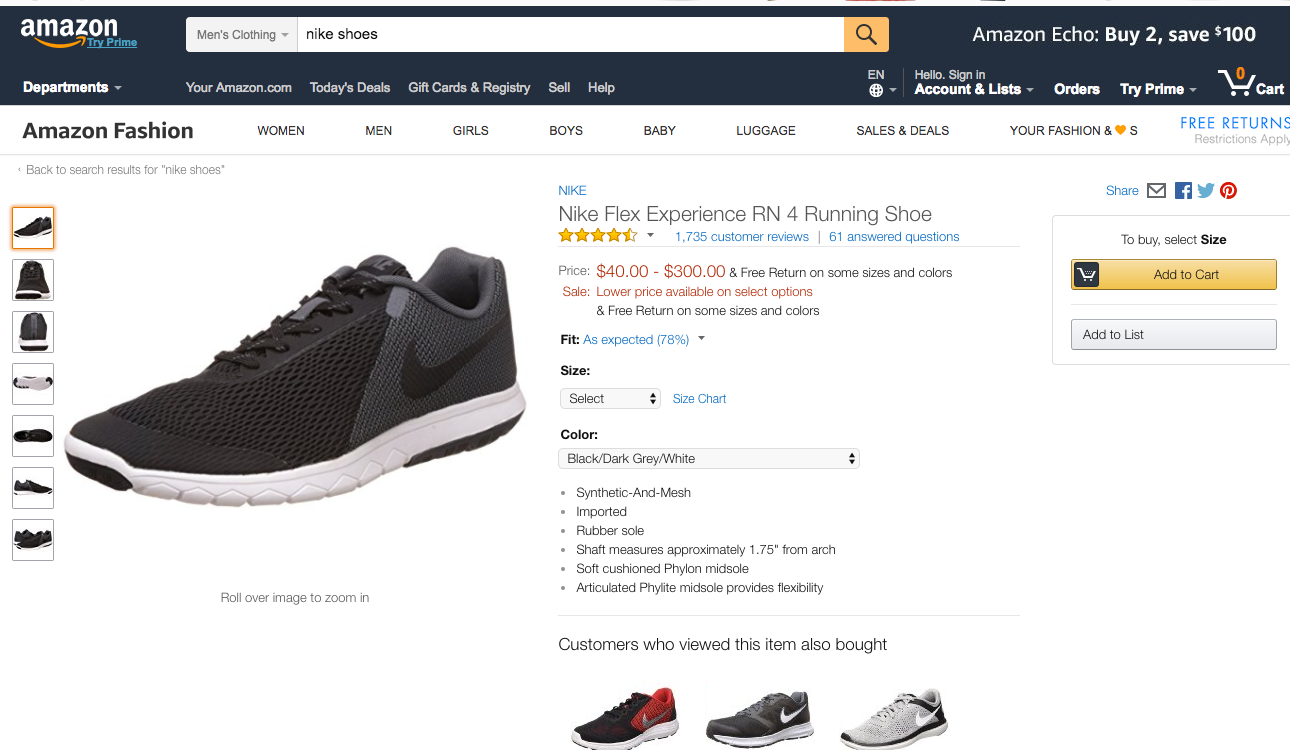This is an image capture from an Amazon.com page, showcasing the "Nike Flex Experience RN4" running shoe listed under men's clothing. The product has garnered a rating of 4.5 stars based on 1,735 customer reviews, with both the rating and the number of reviews displayed in blue text. Additionally, there are 61 answered questions about the product, also highlighted in blue. The price for these shoes ranges from $40 to $300, with an indication in red that a sale is ongoing. It further mentions that a lower price is available on select options, and free returns are available on some sizes and colors.

The main image on the right shows the shoe’s design: it features a white sole with certain areas accented in black. The upper portion of the shoe is predominantly black, with a gray heel counter, and a distinctive black Nike swoosh on the back portion. 

Below the product details, there are options to add the item to your cart or to a wish list, with a prompt to select a size before purchasing. The page also includes a section titled "Customers who viewed this item also bought," which features three different shoe recommendations.